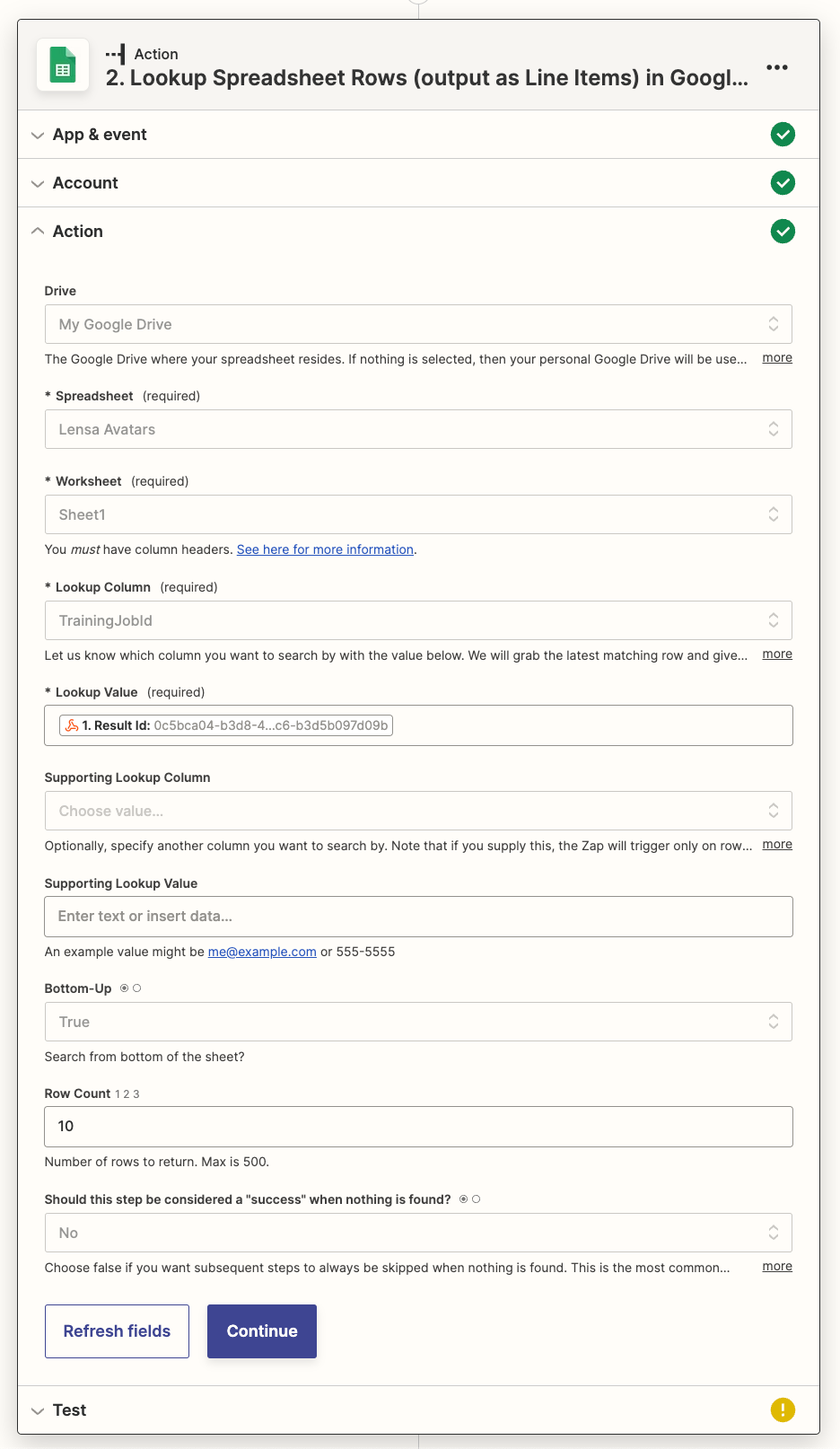The image displays a detailed screenshot of a lookup configuration interface within a Google Sheets integration workflow. At the top, there's a title indicating the step name: "Lookup Spreadsheet Rows." Below that, it specifies the action as "number two," describing it as "Lookup Spreadsheet Rows output as line items in Google Sheets."

The interface is organized into several sections:

1. **App and Event Section**:
    - Displays options for selecting the app (Google Sheets) and the type of event (Spreadsheet Lookup).

2. **Account and Action**:
    - Prompts the user to select their Google Drive account. If no specific drive is selected, it defaults to the user's personal Google Drive.

3. **Spreadsheet and Worksheet Areas**:
    - Fields for selecting the specific Google Spreadsheet and Worksheet where the data resides.

4. **Lookup Parameters**:
    - **Lookup Column**: Specifies the column to search within.
    - **Lookup Value**: Defines the value to search for within the specified column.
    - **Supporting Lookup Column and Value**: Additional fields to refine the lookup criteria.

5. **Additional Settings**:
    - **Bottom Up**: An option to search from the bottom up.
    - **Row Count**: Indicates the number of rows to return, with a maximum of 500. Currently set to 10 rows.
    - **Success Condition**: A checkbox to determine if the step should be considered successful when no records are found. The default option helps subsequent steps to be skipped if nothing is matched, indicating common usage.

6. **Action Buttons**:
    - **Refresh Fields**: A button to update the field options.
    - **Continue**: A navy-colored button to proceed with the configuration.

The user is provided guidance through each step, ensuring an efficient setup for retrieving relevant rows from a Google Spreadsheet based on specified criteria.